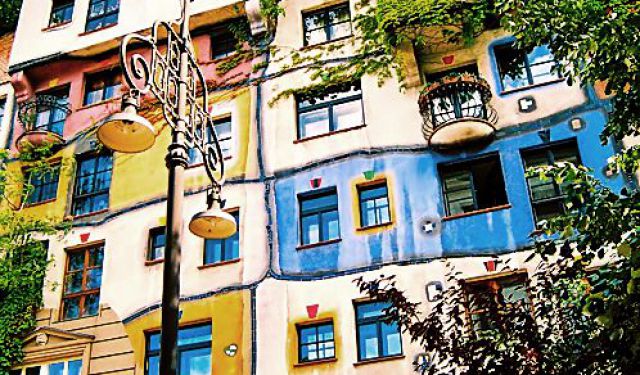A vibrant and colorful building dominates the image, revealing a modern structure with numerous rectangular and square windows. The facade is a mosaic of multicolored sections, featuring striking hues of yellow, blue, red, and white that make each row of the building visually distinct. The scene is enriched with natural elements; a very tall, green tree stands majestically on the right, while another equally tall tree is positioned on the left against the building. A detailed lamppost on the left, painted in brown, showcases intricate iron rodwork adorned with a wired bell decoration, from which two lamps hang symmetrically. Additionally, vine work and a small, protruding balcony add to the architectural charm of the building. The perspective of the image suggests it’s a photograph taken with an upward angle, further stylized with a filter to accentuate the vivid colors, giving it an almost painterly quality.